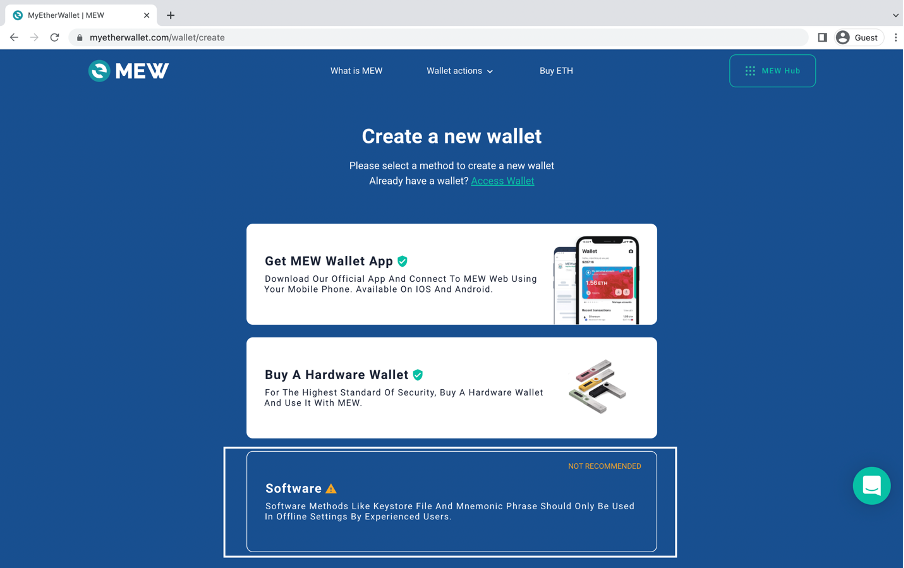This is a detailed screenshot of a web browser displaying a single tab opened to the URL "myetherwallet.com." On the left side of the browser's navigation bar, there are three icons: a back button, a forward button, and a refresh button. On the right side of the navigation bar, there's a pill-shaped button labeled "Guest," followed by a default avatar icon.

The website itself features a predominantly blue background. At the top left corner of the page, the abbreviation "MEW" is displayed next to a green circle icon, which is part of the website's logo. The top navigation menu is divided into three sections: "What is MEW," "Wallet Actions," and "Buy ETH." On the far right, there's a green box labeled "MEW Hub."

Overall, the interface is clean and purposeful, with easy access to essential functionalities and navigation options.